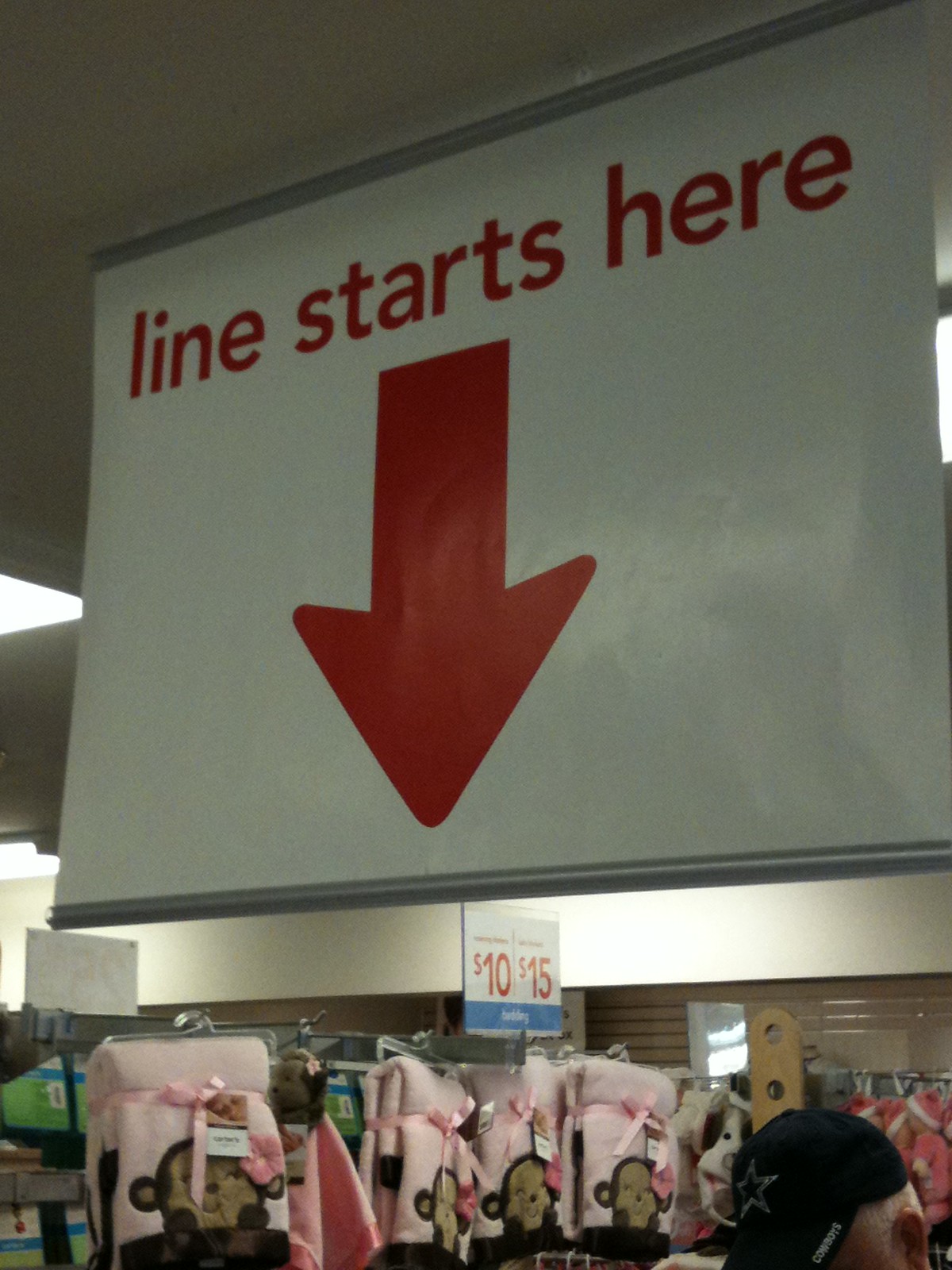In this detailed image captured inside a clothing store, the background is adorned with several racks filled with baby blankets, prominently priced at $10 and $15. The far wall is painted in a beige hue, accompanied by a contrasting white panel. The ceiling overhead is a functional drop ceiling, outfitted with bright fluorescent lights that illuminate the space. In the bottom right-hand corner, the top of a gentleman's head is visible, distinguishable by his blue Dallas Cowboys hat. Dominating the center of the composition is a white ceiling-hung sign with vivid red lettering that reads "Line Starts Here," accentuated by a red arrow pointing downward.